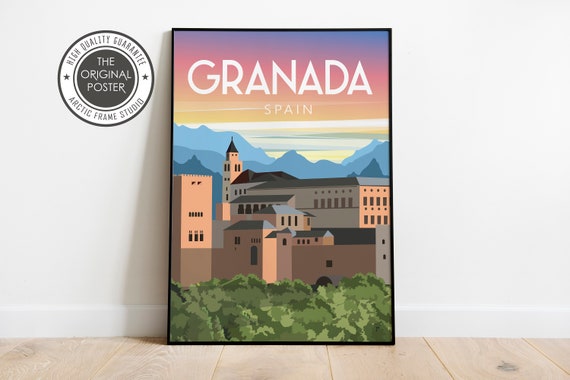The image features a detailed, framed drawing propped against a white wall with a wooden floor. The top of the drawing prominently displays the text "Granada, Spain" in white letters. In the background, a stunning sky showcases a rich mix of peachy pink, lavender, blue, orange, yellow, and white hues, suggesting a vibrant sunset. Beneath this colorful sky, blue mountain ranges, some pointed and some flat, create a serene backdrop. The foreground of the drawing depicts a collection of beige and rust-colored buildings, including churches and castles, with gray and black roofs and a prominent steeple. Green plants adorn the lower part of the scene. In the top left corner of the image, within a circle, it reads "High Quality Guarantee, Arctic Frame Studio, The Original Poster." The artwork is encased in a thin black frame, enhancing its detailed and scenic portrayal of Granada, Spain.